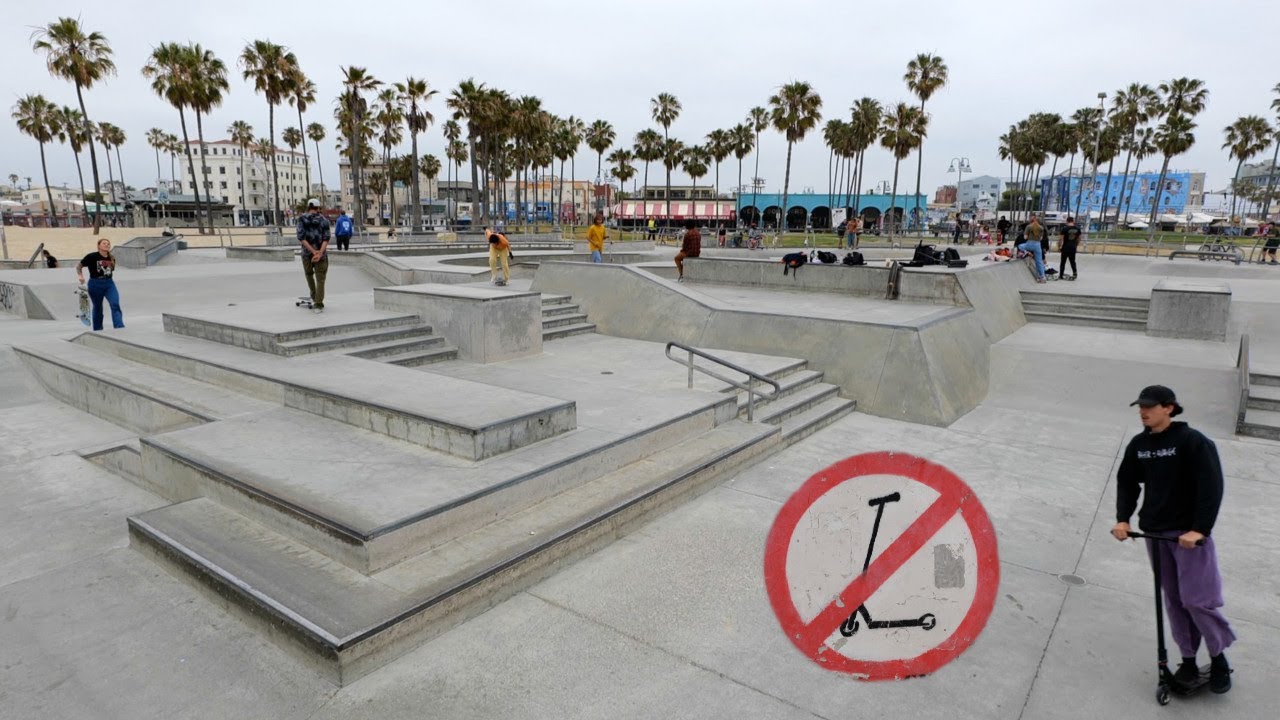In this vibrant outdoor scene, a bustling skate park teems with activity. Skaters and scooter riders alike navigate the various levels, steps, and railings designed for tricks. The park itself is predominantly black with a seamless, sleek concrete design that invites action. Prominently positioned in the bottom center of the image is a large red circle with a diagonal line through the image of a scooter, clearly indicating "no scooters." Nevertheless, a man defies the sign, riding a scooter or a Segway on the right side of the image, distinguished by his black sweatshirt, black cap, and grey trousers.

The backdrop is spectacular with a line of lush palm trees that swing into view, hinting at a temperate climate. Behind them, a mix of buildings peeks through, ranging from potential hotels to restaurants, denoting a lively urban setting. The blue expanse of either a water body or an arch-like structure also catches the eye on the right side of the image.

Among the skaters, one boy on a scooter is noted in the background alongside another with a skateboard, creating a dynamic scene of movement and leisure. The sky hovers with hints of blue, while the diversity of colors captured in the image—ranging from reds and purples to greens and pinks—adds to the vibrant energy of this outdoor skate park, possibly located in a stylish and modern district of Ports.